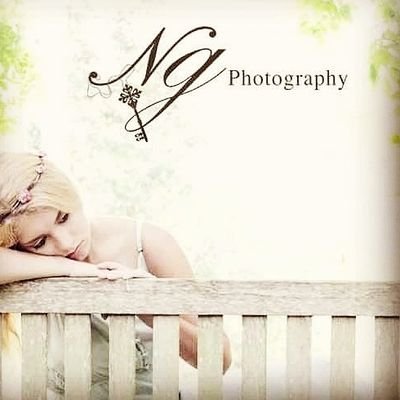The image is a meticulously crafted logo for NG Photography, showcasing a blend of graphic elements and a photograph of a female subject. The square-shaped image features a white, wooden fence with vertical slats and a horizontal bar, extending across the bottom of the visual. On the left side of the fence, a blonde white woman is leaning over it, with her right arm and head resting on the top bar. The woman, who appears somewhat melancholic, is adorned with a floral tiara composed of pink and green elements and wears a light grey-beige dress with bare shoulders and a strap over one shoulder.

In the upper part of the image, the text "NG Photography" is prominently displayed. The "NG" is rendered in luxurious cursive script with a black key weaving through the loop of the 'G,' while the word "photography" is printed in a simpler, smaller font. The key is centered to the left, beneath the NG text. The background features a predominantly light beige tone with subtle green leaves in the upper left and right corners, adding a touch of nature to the otherwise clean and simple composition. A faint drop shadow around the edges of the image lends depth to the overall design, enhancing its professional and polished appearance.